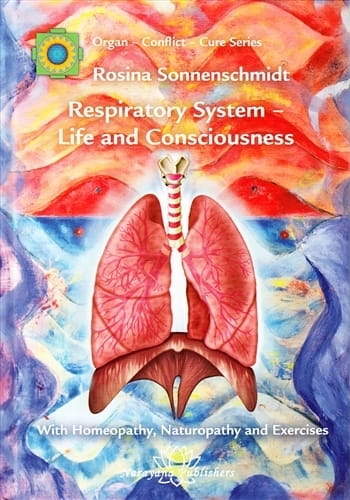The image appears to be a vividly colorful cover, likely for a pamphlet or book, with a mix of swirly patterns in red, white, blue, purple, pink, and notably orange at the top blending into blue at the bottom. The central theme is organ donation or health, depicted with a stylized human skeleton on a blue background. The upper section features oranges and yellows highlighting the ribcage, transitioning to blues accentuating the lower ribs and bones. Superimposed on this skeletal structure are bright, detailed illustrations of organs such as lungs, possibly kidneys, with visible veins in reds and browns.

At the top left corner, a distinctive green logo is present, containing green rectangles flanking a yellow scalloped circle, which encases a black circle further encircling a blue circle with white accents. The title at the center top reads "Organ Conflict Cure Series" in white upper and lower case letters, followed by the author's name, "Rosina Sonenschmidt." Below that, it states "Respiratory System," and further down, "Life and Consciousness," all in white text. The bottom part of the cover features the tagline "With Homeopathy, Naturopathy, and Exercises," indicating the holistic nature of the content, emphasized by a colorful representation of the lungs and possibly other organs.